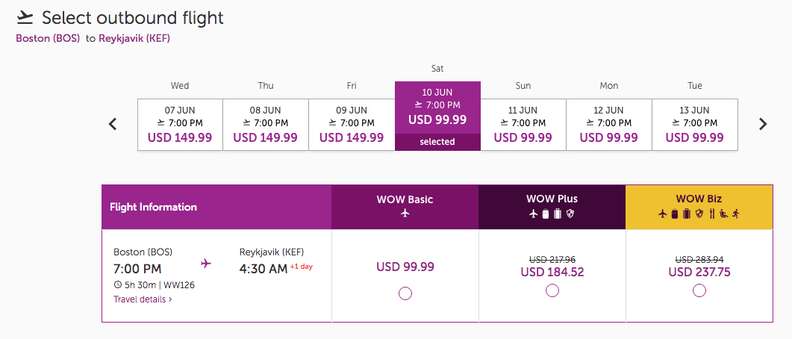The image depicts a section of a flight booking website featuring a selection of outbound flights. Prominently displayed is an airplane graphic alongside the words "Select Outbound Flight." The route shown is from Boston (BOS) to Reykjavik (KEF).

Below this header, a timeline reveals available flight options, all scheduled for 7 p.m., with corresponding prices:
- Wednesday: $149.99
- Thursday: $149.89
- Friday: $149.89
- Saturday: $99.99 (highlighted in purple, indicating it is the selected flight)
- Sunday: $99.99
- Monday: $99.99
- Tuesday: $99.99

Flight information specifies the departure from Boston (BOS) at 7 p.m. and arrival in Reykjavik at 4:30 a.m. the following day. A note in orange mentions that the flight spans over one day.

Different fare classes are detailed with prices:
- Wow Basic: $99.00
- Wow Plus: $184.52 (discounted from $217.00)
- Wow Biz: $237.75 (discounted from $283.94)

The "Travel Details" section is clickable and highlighted in purple for further information.